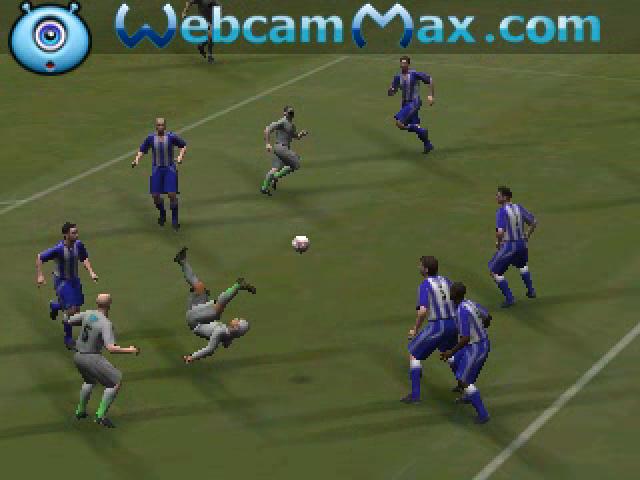This detailed and cleaned-up caption consolidates the critical elements from each voice description:

In this computer-generated screenshot of a video game, the scene depicts an intense soccer match. At the top of the image, "webcammax.com" is displayed in light blue and dark blue font. Near the 'W' of "webcammax.com," there is a small blue alien with a single eye featuring a blue iris and black pupil, two antennae, and an open mouth showing a red interior. The soccer field hosts two distinct teams: one in blue and gray vertical striped tops with blue shorts, and the other in all gray with green socks and green lettering on their jerseys. There are six players from the blue team and three from the gray team visible. Among them, a gray team member is dramatically mid-flip, executing a bicycle kick with his back parallel to the ground while striking a white and red soccer ball. The referee, dressed entirely in black, can also be seen in the background overseeing the action.